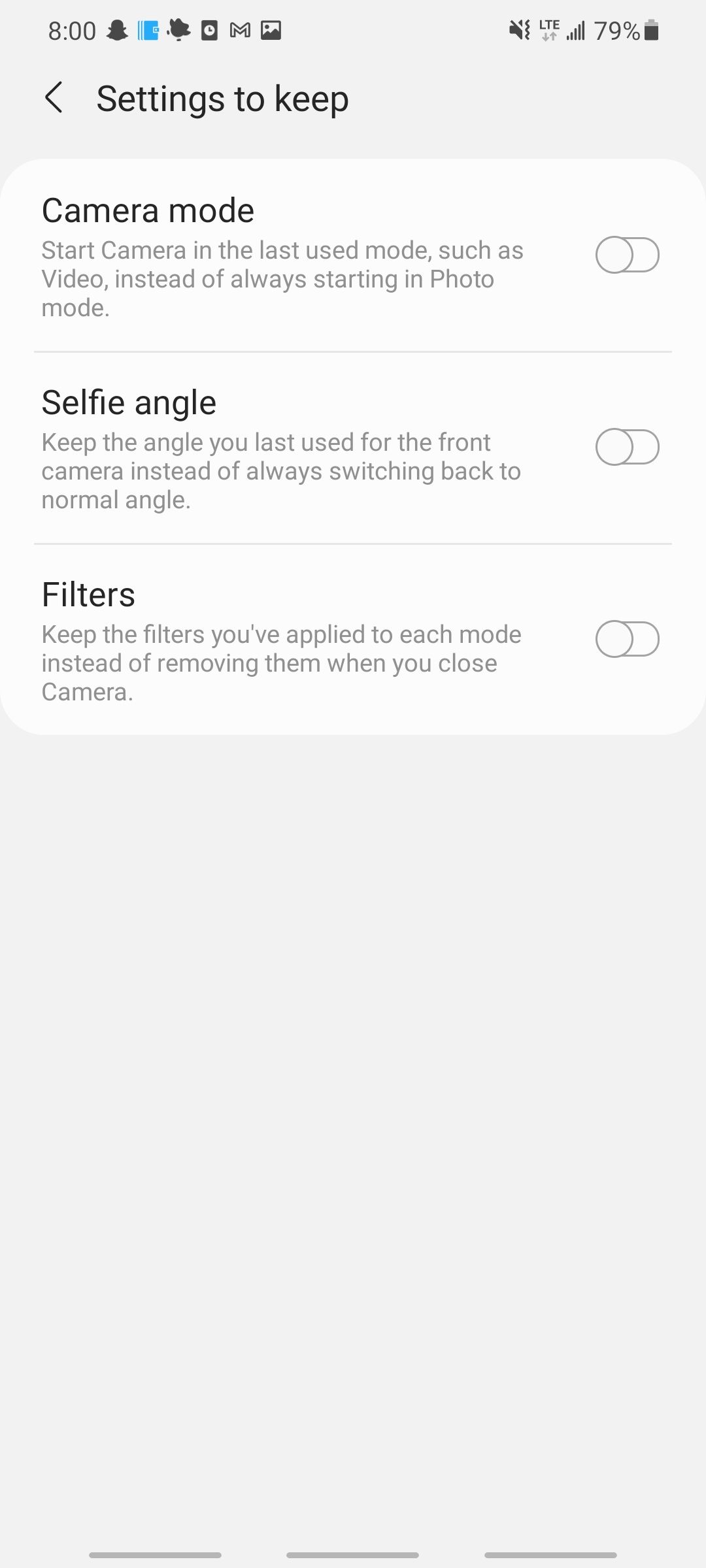This image is a screenshot of a smartphone in incognito mode with a light gray background. At the top, the status bar indicates the time as 8:00, and includes several icons: one each for incognito mode, time, Gmail, Google Photos, sound (which is off), LTE connectivity, and a battery level at 79%. Below the status bar, there is a left-facing arrow and a "Settings to keep" tab.

The main section of the screen is divided into vertical entries with specific settings options:

1. **Camera Mode**: This setting allows the camera to start in the last used mode, such as video, instead of always defaulting to photo mode. The current status is off.
   
2. **Selfie Angle**: This setting enables the front camera to keep the angle you last used, rather than switching back to the normal angle by default. This option is currently off.
   
3. **Filters**: This setting permits filters applied to each mode to be retained instead of being removed when the camera is closed. This option is also off.

At the bottom of the screen, there is a gray section with three horizontally aligned buttons, each designated by three gray lines. The screenshot captures a settings tab on a smartphone device, detailing various camera settings and their current statuses.